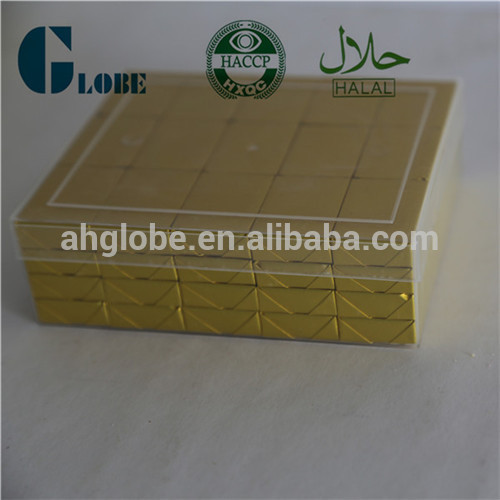The photograph depicts a clear acrylic box with a matching lid, resting on a white surface. Inside the box are numerous gold-wrapped rectangular bars, each individually packaged. The arrangement is precise, with four columns and five rows, each stack containing four layers, totaling 60 bars. On the upper left corner of the box, the word "GLOBE" is displayed in blue. The center of the image shows a circular green logo encompassing an eye, with the text "HACCP" and "HXQC" underneath. To the right of this logo, "HALAL" is written beneath Arabic script, indicating the product is permissible according to Islamic law. Additionally, the website "ahglobe.en.alibaba.com" is printed in white across the center of the image.